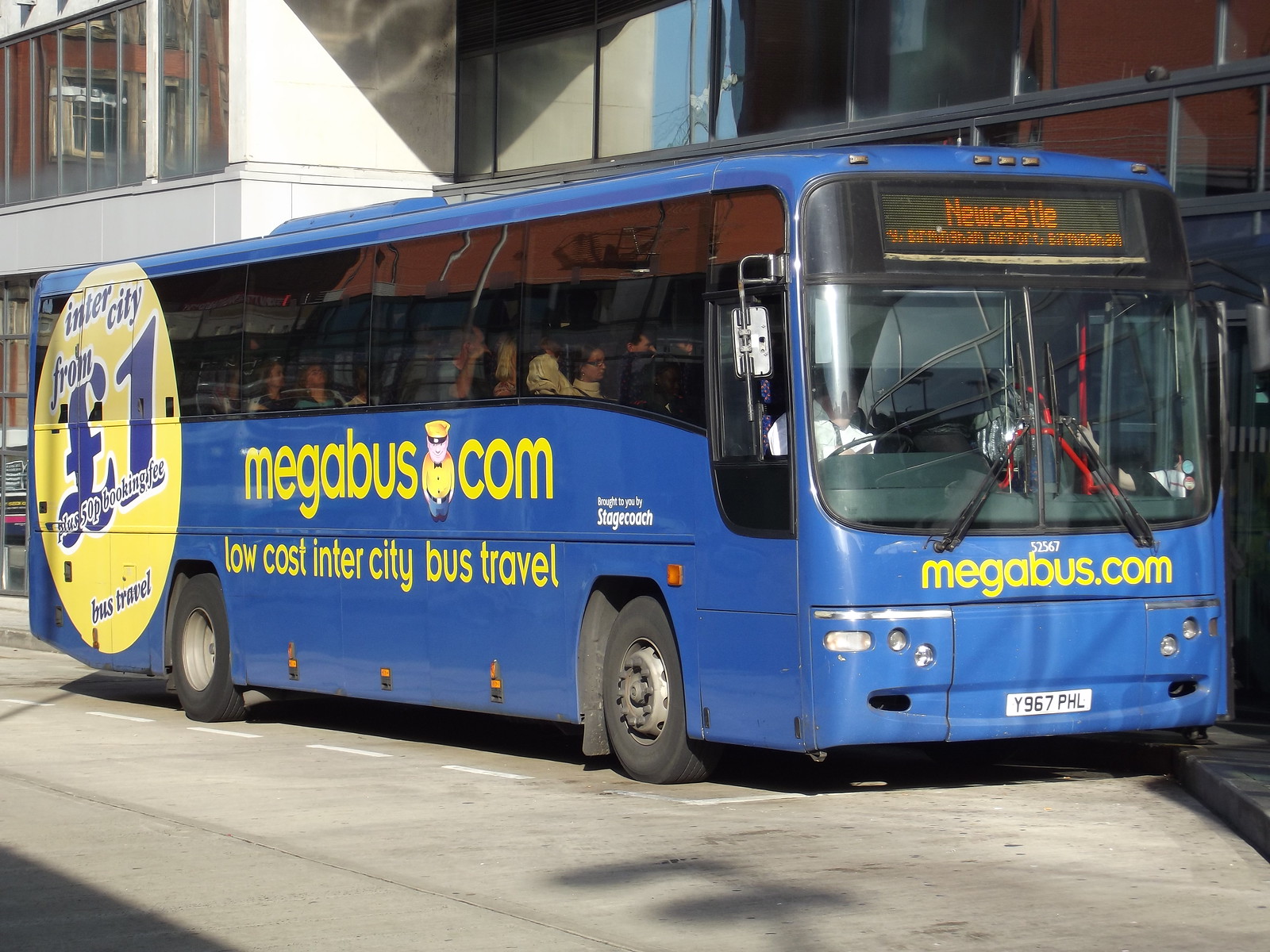This image captures a large, blue and black Megabus parked on a city street with several buildings in the background. The bus's front marquee prominently displays "Newcastle," though the following line is partially legible and suggests "Birmingham Airport." The bus, identified by the number 52567, features the website "megabus.com" in yellow font just below the windshield. The white license plate reads Y967PHL. It is parked within a marked area outlined by white dots, which likely indicate designated bus parking.

On the side, bold yellow lettering spells out "megabus.com" below the windows, along with the tagline "low-cost intercity bus travel" underneath. The rear section of the bus displays a large yellow graphic that stretches from top to bottom, containing the partial slogan "inner city from L1 plus," with the concluding phrase "bus travel" plainly visible. There is also a note in small white font on the right side reading "brought to you by stagecoach." The tinted windows provide a glimpse of passengers seated inside, suggesting the bus is in use. The building adjacent features white and red windows, adding an urban backdrop to the scene.